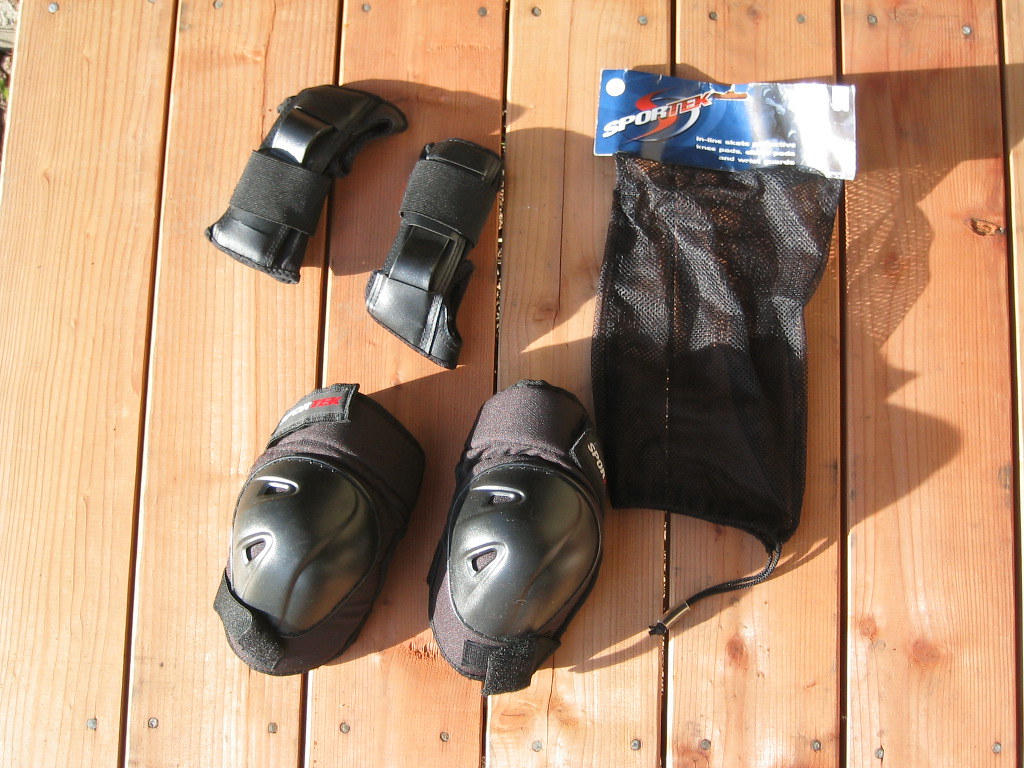This photo is a detailed top-down view of a set of black protective gear, laid out on a light wooden deck, likely outdoors in direct sunlight. Positioned in the bottom left-hand corner are a pair of black knee pads, with hard plastic exteriors and velcro straps for securing them around the legs. In the top left-hand corner are a pair of black wrist guards, also featuring velcro straps. To the right of these items is a black mesh bag meant for storing the protective gear. The mesh bag is unopened and has a cardboard label at the top that reads "Sportek" and "inline skate protective knee pads and wrist guards." The deck surface appears to be composed of treated boards, indicating its outdoor setting. This meticulously arranged photograph seems intended to advertise the athletic gear for sale, highlighting the knee pads, wrist guards, and storage bag as a complete set.